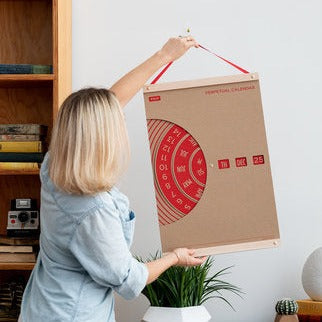In this photograph, a Caucasian woman with shoulder-length blonde hair is preparing to hang a unique, vertically rectangular calendar on a white wall. The calendar, resembling the color of unstained cardboard or a shopping bag, features a distinctive semicircular cutout on the left edge, exposing concentric circles that can be turned to adjust the date. The right side of the calendar houses three small windows for displaying the year, month, and day, controlled by these turning wheels.

The woman is dressed in a rolled-up, light blue denim shirt. Her left hand holds the calendar by a red ribbon attached at the top. The calendar itself may be constructed from brown wood or colored cardboard and includes intricate details such as a light blue border at the bottom and red dials with numbers.

The setting appears to be her home, marked by a wooden set of shelves on the left edge of the frame and a green potted plant at the bottom, possibly accompanied by a cactus and a white vase nearby. The overall scene captures a moment of home organization with a touch of traditional charm, represented by the manual operation of the perpetual calendar.